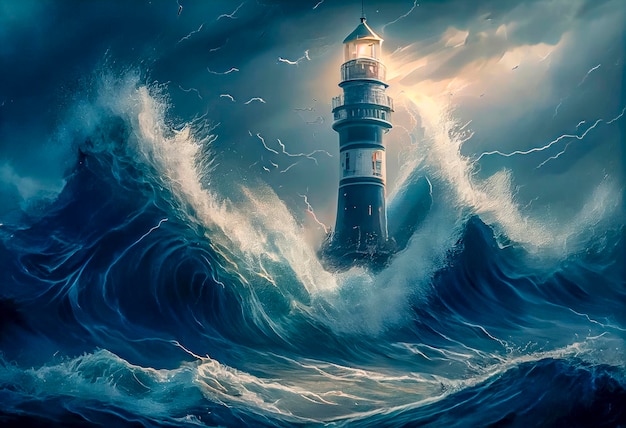This is a highly stylized acrylic painting depicting a lighthouse amidst a fierce storm. The lighthouse, standing approximately 20-30 feet tall, is positioned slightly right of center, its blue cylindrical structure prominently jutting from the turbulent waters. Encircled by massive waves that crash against it, nearly reaching the illuminated glass top covered by a conical blue cap, the lower portion of the lighthouse is obscured by the foamy surf. A white band wraps around its midsection, and a walkway is visible two-thirds of the way up. The scene is dominated by a palette of dark blues, grays, and whites, with the sky and ocean almost blending together in their intensity. There are streaks in the stormy sky, possibly representing lightning, and a faint yellow tinge emanates from the lighthouse's light. The atmosphere is menacing and monochromatic, capturing the raw power of nature. Notably, the painting lacks an artist's signature.